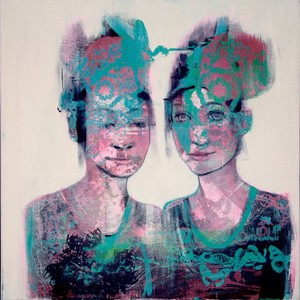This image captures an abstract painting portraying two women standing side by side against a stark white background, likely watercolor paper. The artistic style employs a vivid interplay of pinks, greens, dark blues, and whites, with an emphasis on the facial details of the women. Both women feature intricate facial structures with defined eyes, noses, and mouths, though their bodies lack arms.

The woman on the right tilts her head slightly left, her hair black with a cascade of green paint seemingly poured over her head, flowing past her eyes and nose. Her eyes are strikingly blue, and she is dressed in a red and black top interspersed with green hues.

The woman on the left turns her head rightward, her eyes smaller and darker compared to her counterpart. She, too, has green paint dripping down her face and onto her dress, which appears darker with tones of black, blue, and green. Above them, the colors—especially greens and pinks—burst in a splotchy, explosive manner, adding to the abstract essence of the piece.

This evocative artwork, reminiscent of an Andy Warhol print, is marked by its low-resolution capture, adding a degree of obscurity to its vibrant and contrasting visual presentation.